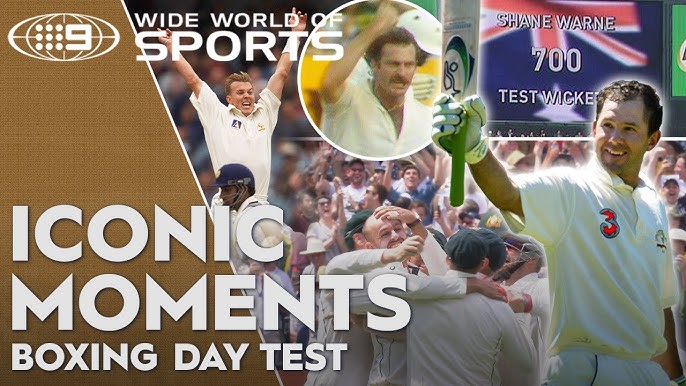The image is a vibrant collage featuring several sports scenes overlaid to create a single, dynamic composition. At the bottom left corner, bold white text reads "Iconic Moments Boxing Day Test," while at the top left, the text "Wide World of Sports" is prominently displayed. Towards the bottom right, more detailed text, "Boxing Day Test," highlights the event.

Front and center, a cricket player with wavy dark brown hair, wearing a polo shirt with the number 3, holds a cricket bat in his right, gloved hand, smiling broadly. This player stands out against a backdrop of lively celebration. Just behind him, white text reads "Shane Warne 700 Test Wickets," with the UK flag subtly incorporated into the design.

In the middle of the image, another group of athletes is seen hugging, reveling in their victory. Farther in the background, a man with a fierce, joyous expression is being lifted up, his arms raised in triumph. The scene appears crowded with jubilant fans, predominantly men, all sharing in the excitement and victory, encapsulating the spirit of these iconic sporting moments.